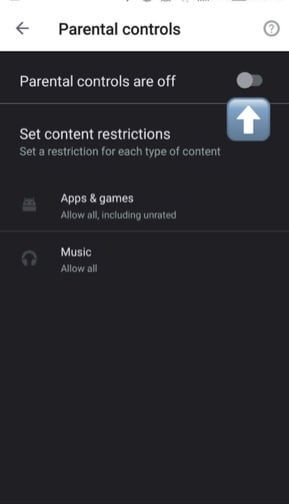The image depicts a section of a website user interface dedicated to parental controls. At the top, there is a thin, gray, angled outline that is partially incomplete, framing the section. Inside this frame, the heading "Parental Controls" is prominently displayed in black text. 

A leftward-pointing gray arrow and a circular icon with a question mark are also present near the heading. Beneath this, a black notification box informs users that "Parental controls are off," written in white letters. Adjacent to this notification, a slider bar is visibly set to the off position.

To the right, there is a blue box featuring a white arrow that points upwards towards the notification. Inside the blue box, the instructions "Set contents restrictions" are provided. Further down, another instruction, "Set a restriction for each type of content," is visible.

The subsequent section lists types of content with corresponding restrictions. For "Apps and Games," a small icon on the left side indicates the category, although it is faint and gray. The accompanying text states, "Allow all, including unrated." Below this, the "Music" category is represented by a headset icon, with the text, "Music all," written in white. The description ends with a blank black space, extending to the bottom of the section.